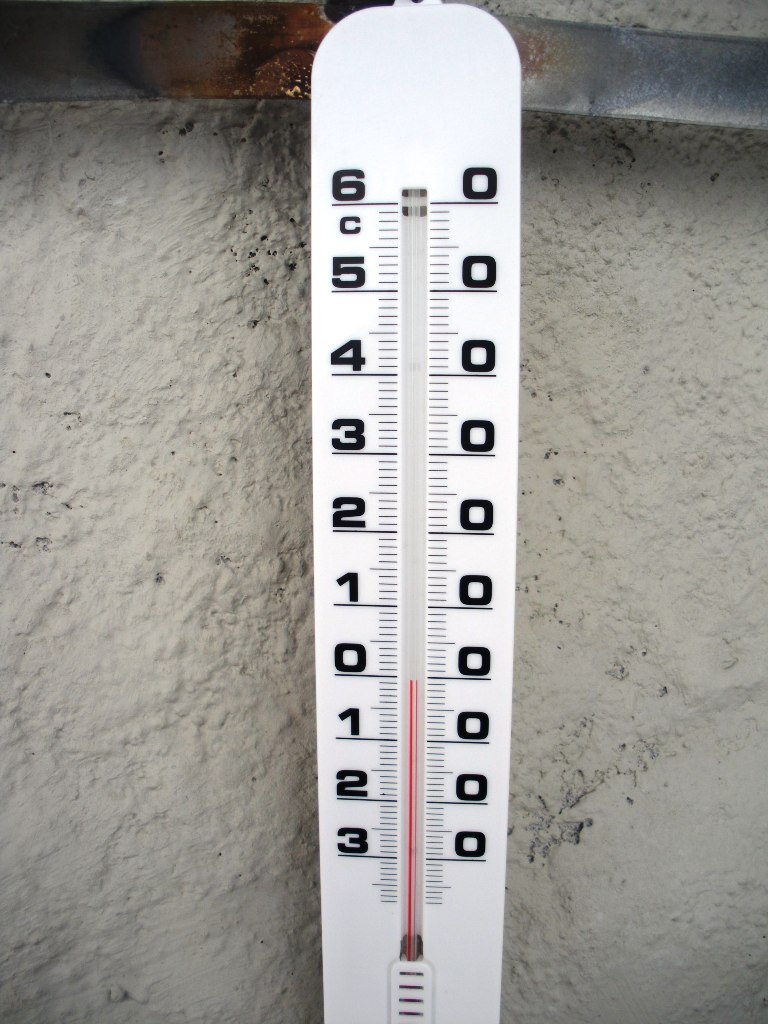This outdoor photograph features a white concrete wall with a thermometer mounted prominently in the center. The thermometer, encased in a white plastic frame, measures ambient temperature in Celsius. Black numerals marked on the thermometer start at the top with 60°C, followed by 50, 40, 30, 20, 10, and 0°C, indicating positive temperatures. Below the 0°C mark, the thermometer shows -10, -20, and -30°C. A thin black line, signifying the Celsius scale, is printed vertically alongside a black "C" for Celsius at the center of the scale. The glass tube at the heart of the device contains a red line that registers the current temperature, precisely at 0°C. In the top left corner of the image, a piece of wood—likely part of a shelf or eave—extends slightly into the frame, providing a touch of contrast to the otherwise stark background.